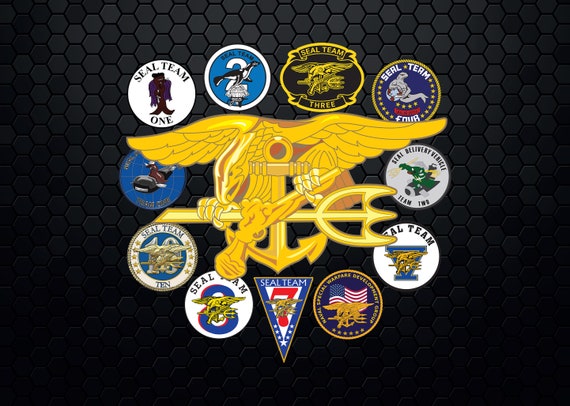The digitally-created image, set against a black background with a hexagon grid pattern, prominently features the Navy SEAL emblem at its center. This emblem is depicted in gold and showcases an eagle with a flintlock pistol in one claw and a pitchfork in the other, all mounted on a gold anchor. Surrounding this central emblem are eleven distinct patches representing various SEAL Teams. These circular patches, except for a triangular one representing SEAL Team 7, display the unique insignias and numbers of each team. Notable patches include SEAL Team 1's white insignia, SEAL Team 2's blue emblem, SEAL Team 3's black patch with yellow lettering, and SEAL Team 4's blue and gray design. Additional patches encompass designs featuring seals, a black whale, the American flag, and references to the Special Warfare Development Group. The image encapsulates the diversity and unity of the Navy SEAL Teams through their distinct yet cohesive insignias, all integrated into a meticulously detailed digital art composition.